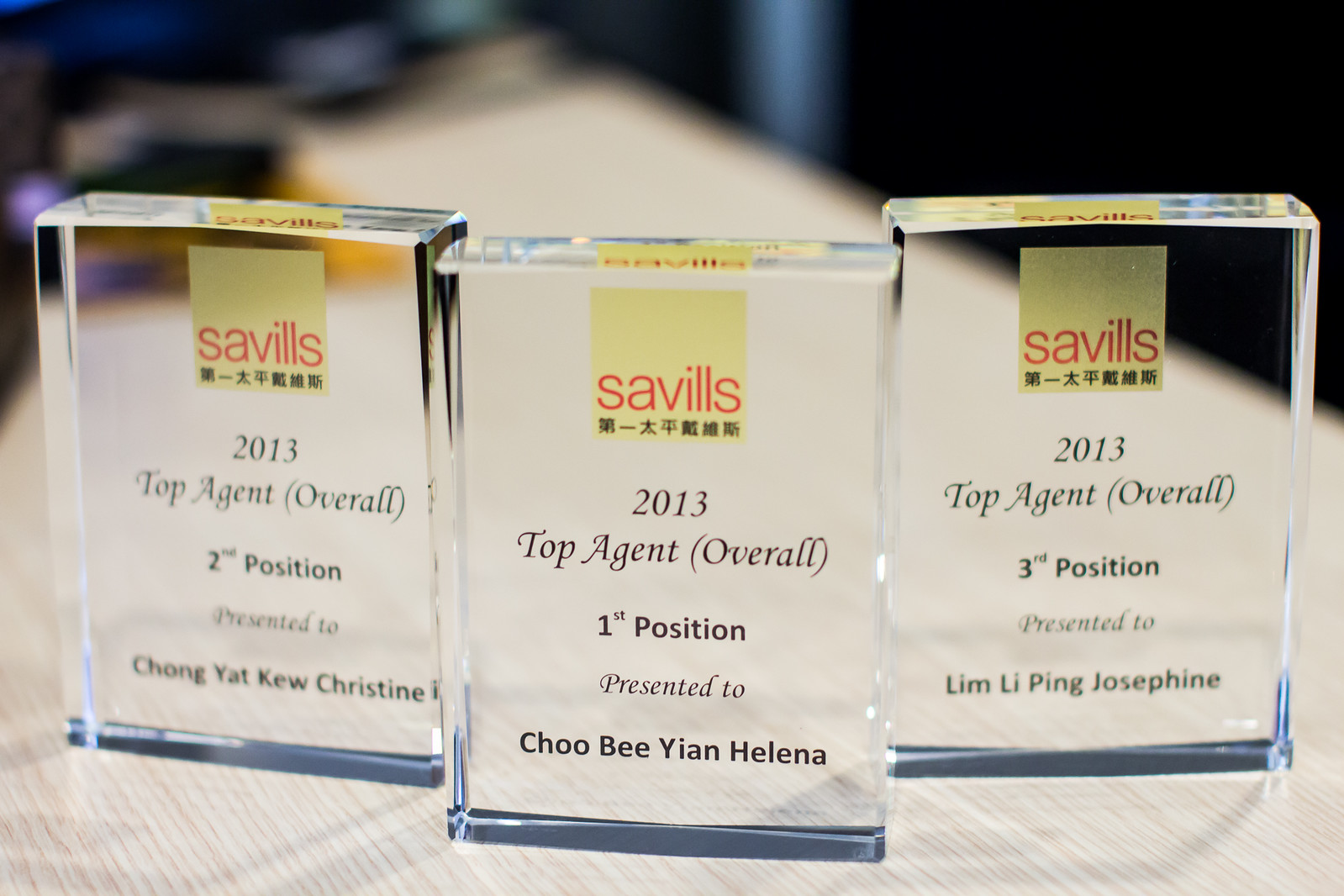The photograph showcases three elegant, glass or transparent plastic rectangular trophies displayed on what appears to be a clean, white or light wooden table. Each trophy features a uniform design with a distinctive gold square at the top center, containing red letters that read "Seville's" and Asian characters underneath. Below this logo, in black letters, the inscription reads "2013 Top Agent Overall." The leftmost trophy is for the Second Position, presented to Chong Yat Kew Christine. The center trophy signifies the First Position, awarded to Chu Bi Yin Helena. The rightmost trophy represents the Third Position, given to Lim Lee Ping Josephine. The background of the photo is blurry and dark, causing the trophies to prominently dominate the foreground.